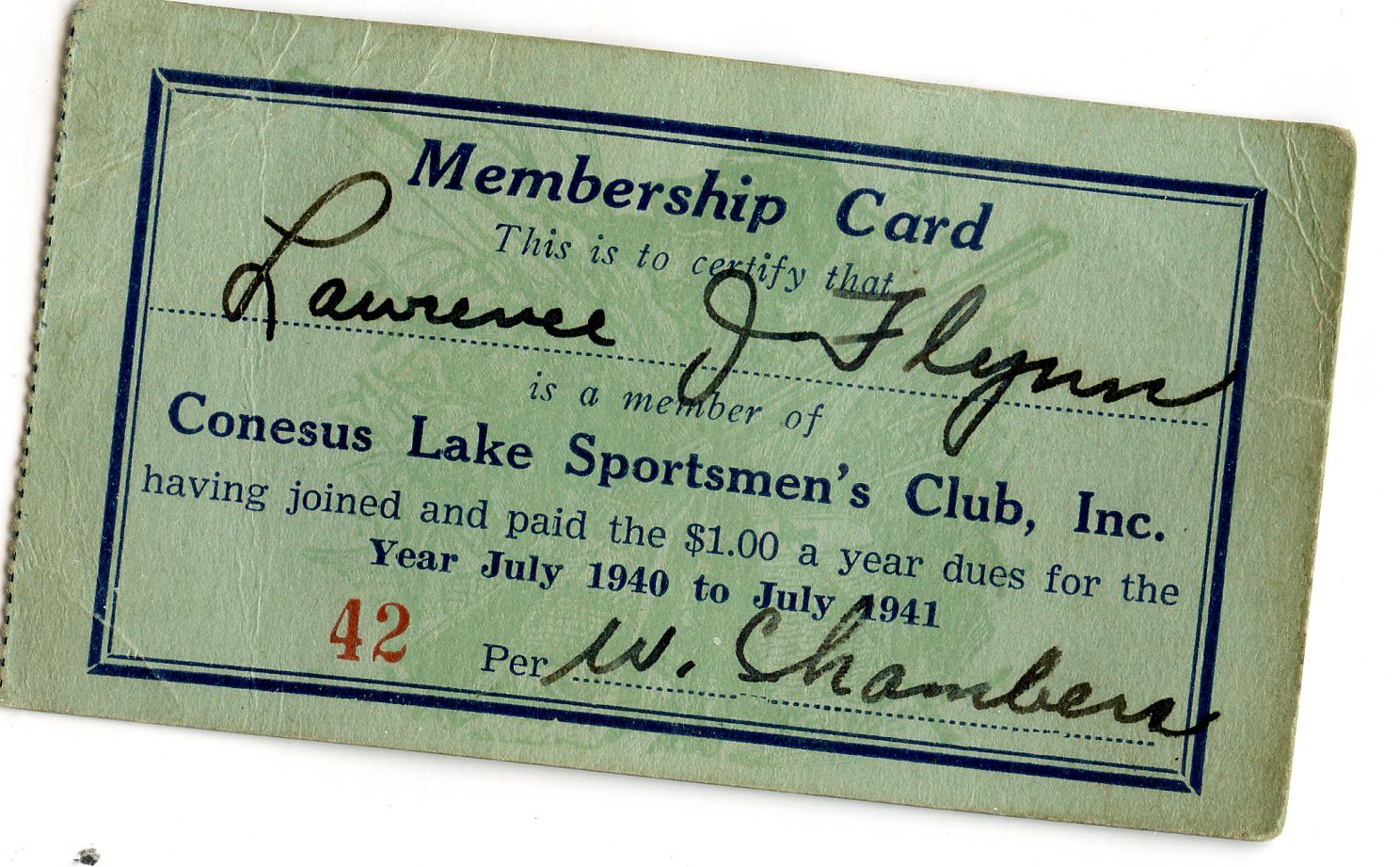In this photograph, an older membership card for the Canesis Lake Sportsman's Club, Inc. is slightly off-center, tilted from left to right. The card, greenish and wrinkled from being kept in a wallet, shows signs of wear with a slightly torn, variegated left edge. The text certifies Lawrence J. Flynn as a member of the club, having paid the $1 annual dues for the period from July 1940 to July 1941. The membership card, designated with the number 42 in red letters, is signed in black ink by W. Chambers. The card also features a black and blue border, with most of the text in blue, capturing a sense of its historical and well-preserved condition despite its age.